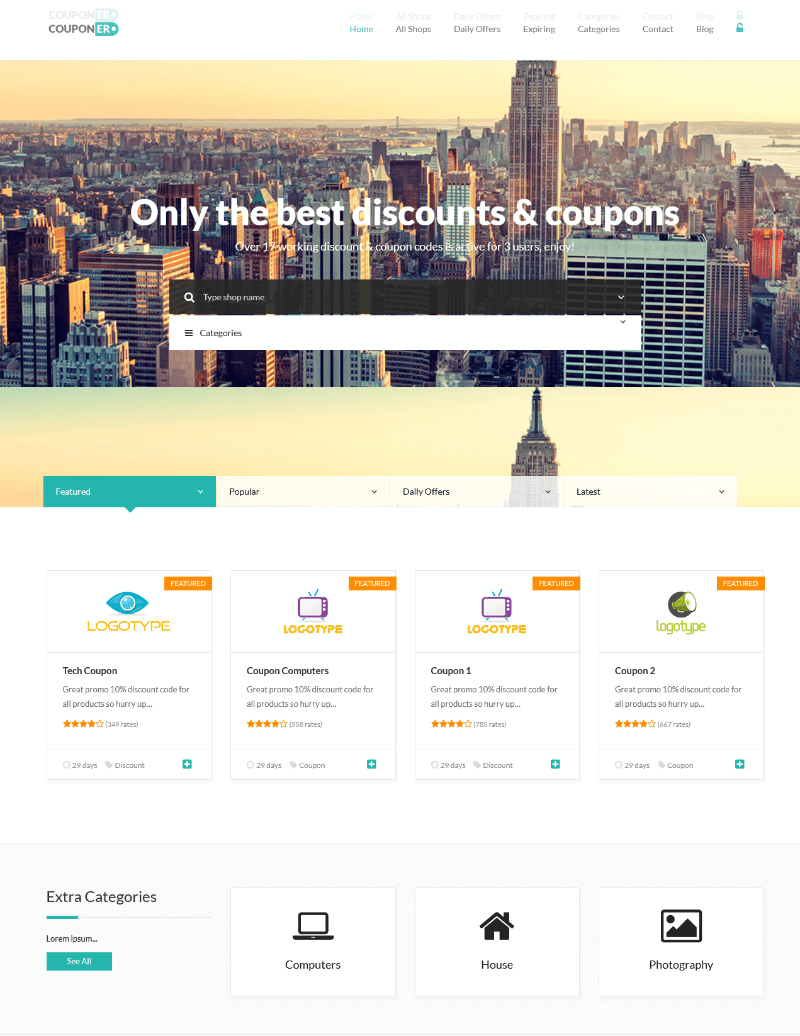This is a detailed webpage design for a coupon website named "Coupon ER." The site is primarily taller than it is wide, resembling the appearance of a computer screen. At the very top, the logo features the text "Coupon ER," with the "ER" enclosed in a half oval. The logo sports a teal color scheme, with "ER" in white font and "coupon" in black. An identical, slightly faded logo is superimposed above the original for a shadow effect.

The navigation menu includes the following items: Home, All Shops, Daily Offers, Expiring Categories, Contact, Blog, and a lock icon, which likely indicates a secure login or account area.

The main background image is a cityscape with a river visible on the right side. Below this focal image is a list of various coupons offered by the website. Each entry in the list is labeled "Logotype" and features a specific coupon name along with some descriptive text and star ratings. The first coupon is "TechCoupon," followed by "Coupon Computers," "Coupon 1," and "Coupon 2."

At the bottom of the page, there is a box containing additional categories. Despite the Latin placeholder text ("Lorem ipsum") indicating ongoing development, the categories currently listed are Computers, House, and Photography. These sections are likely intended to be populated with relevant content once development is complete.